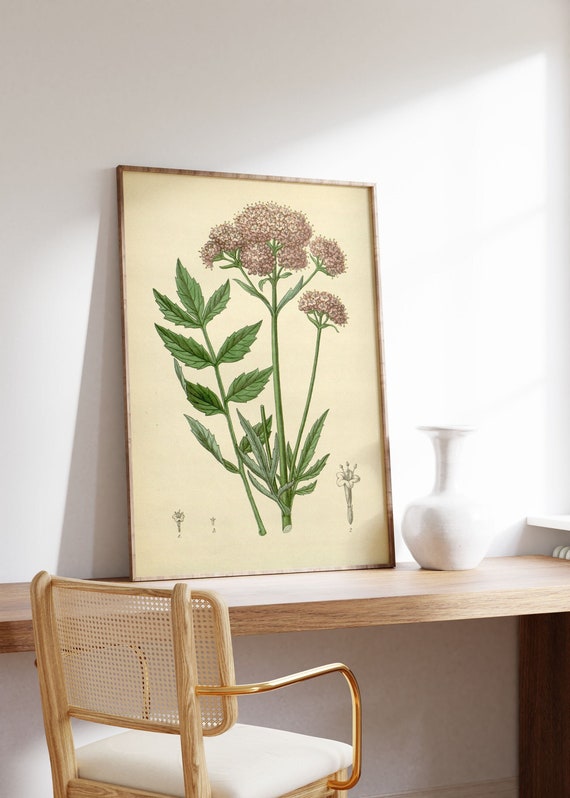The image depicts a sunlit room with beige and off-white tones, featuring a corner area with a built-in wooden counter or desk. Central to the composition is a rectangular drawing or illustration of a flower plant on an off-white background, framed by a very thin wooden border. The artwork leans against a stark white wall, partially resting on the counter. The depicted plant has green leaves and pinkish flowers, consistent with what one might find in a biology book, with a notable frond of leaves extending from the left. Among the additional illustrations at the bottom of the frame are smaller flowers and leaves. To the right of the artwork on the counter sits an off-white vase, its presence accentuated by subtle shadows. Positioned in front of the counter is a chair characterized by rounded metallic brass arms, a white cushioned seat, and a wicker cane back supported by light tan wood. The setting, possibly part of a home or office, combines elements of natural wood and muted tones to create a serene, functional space.